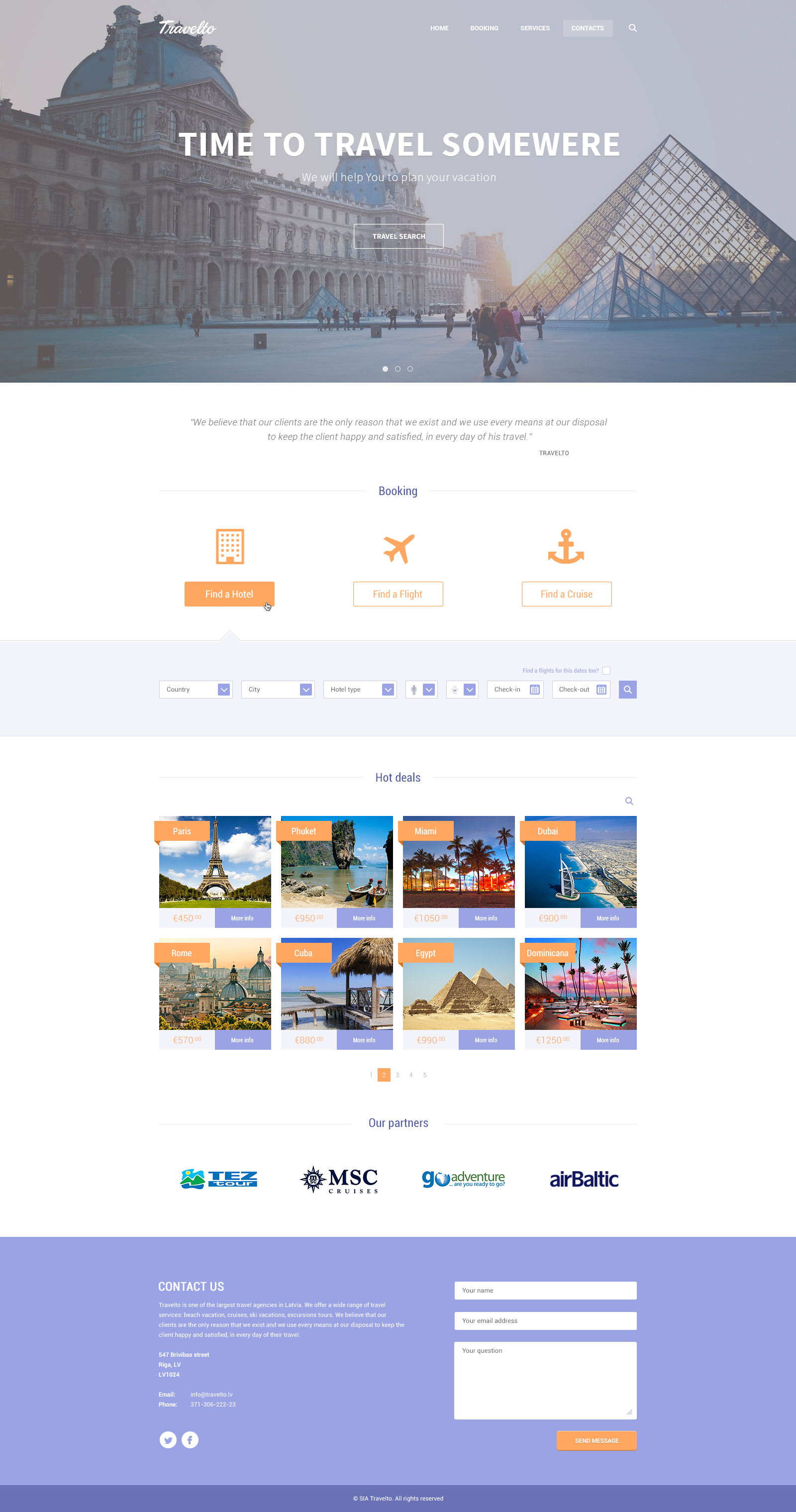A vibrant and bustling scene unfolds in this outdoor photograph taken at the iconic Louvre Museum in Paris. Dominating the background is the historic Louvre Palace, its classic tan stone architecture beautifully juxtaposed with the modern glass pyramid that stands prominently in the museum's courtyard.

Overlaying the image is a variety of unidentifiable white text at the top left and right corners. Prominently, the phrase "Time to travel somewhere" is displayed in crisp white lettering just below. Beneath this, more white text that is too blurred to decipher appears, along with a white space containing gray, indistinguishable text.

In the foreground, an image of an orange building, an airplane, and an anchor symbolize various travel-related elements such as accommodations, flights, and sea voyages. A blue background enhances these icons, adding a dynamic contrast to the scene. Below this, several white drop-down menus featuring black text are visible but not readable.

To the right, a white section features the phrase "Hot Deals" in faint black text, drawing attention amidst the surrounding visuals. This portion blends seamlessly with an illustrative compendium of world landmarks, including the Eiffel Tower in Paris and the Great Pyramids of Egypt, reflecting the expansive spirit of travel.

Company logos in black appear alongside these elements, while a large blue bar containing white text stretches across part of the image. Further right, three input fields hint at functionality for user interaction: spaces for a name, email address, and a note, accompanied by an orange "Submit" button.

The composition concludes with a darker blue section at the bottom, embedded with more unreadable white text, framing the image with a sense of completion yet urging viewers to take action.

This detailed collage fervently encapsulates the allure and practicality of travel, beckoning adventurers worldwide to embark on their next journey.